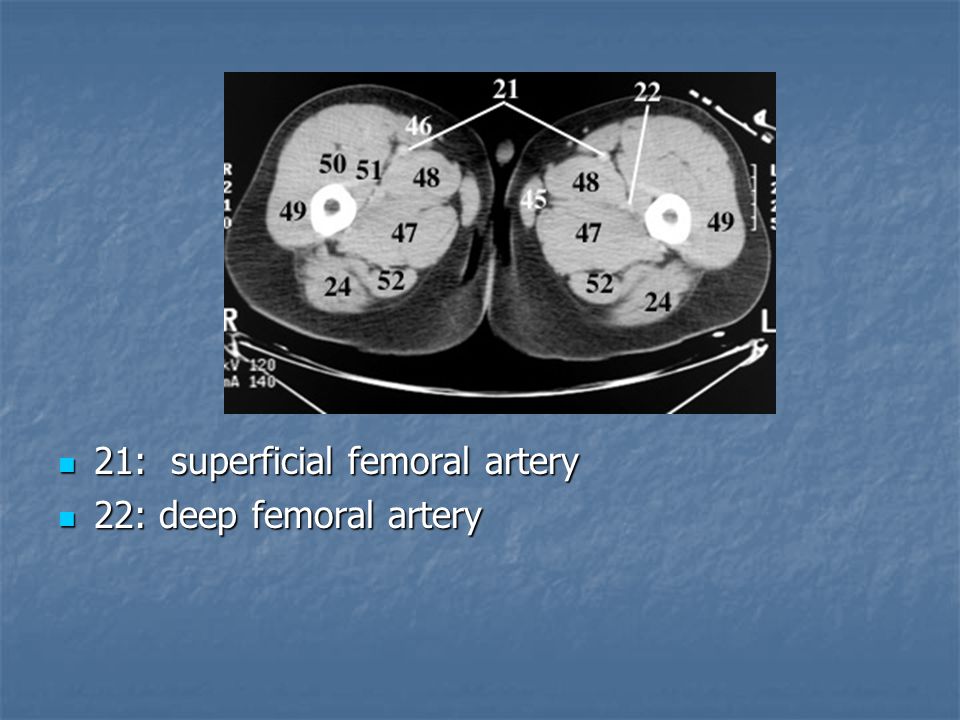The image appears to be from a medical textbook or a PowerPoint presentation featuring anatomical structures, specifically a cross-sectional view of the human thigh. It is set against a blue background, which might be a slide design or a blue surface where an informational card sits.

At the top of this blue background is a black card, occupying about a quarter of the space, that displays two circular cross-sections side by side, presumably representing an X-ray or MRI image. The cross-sections are labeled with various numbers indicating different anatomical parts. The labels include 21 (superficial femoral artery), 22 (deep femoral artery), along with other numbers like 46, 45, 50, 51, 48, 49, 47, 24, and 52. These numbers likely correspond to specific tissues or structures within the image, with pointers linking them to their respective parts.

Both cross-sections contain a white circle with a dark center, reminiscent of cell depictions in biology. A white "R" and "L" are noted below the image, marking the right and left sides of the cross-section, emphasizing the orientation typically seen in radiographic images. Beneath the anatomical illustration, text bullets clarify that number 21 denotes the superficial femoral artery and number 22 signifies the deep femoral artery, offering further explanation of the pictured structures.